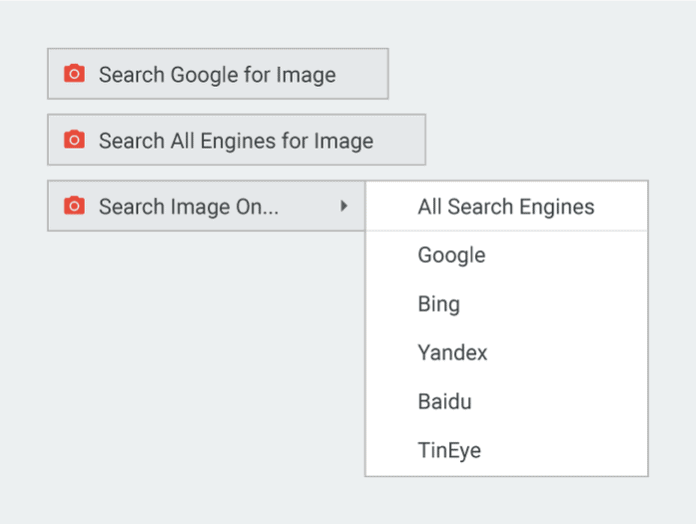In this image, we see a screenshot depicting an interface for image searches. The main screen features a light blue background with three selectable buttons, each marked by a red camera icon followed by a search option. The first button reads "Search Google for image," the second states "Search all engines for image," and the third says "Search image on..." with an arrow pointing to the right.

Superimposed on this main screen is a white pop-up window listing six search engine options. These choices are as follows: 
1. All search engines
2. Google
3. Bing
4. Yandex
5. Baidu
6. TinEye

The interface is designed to allow users to perform image searches using various forms, seamlessly offering the option to use multiple search engines.